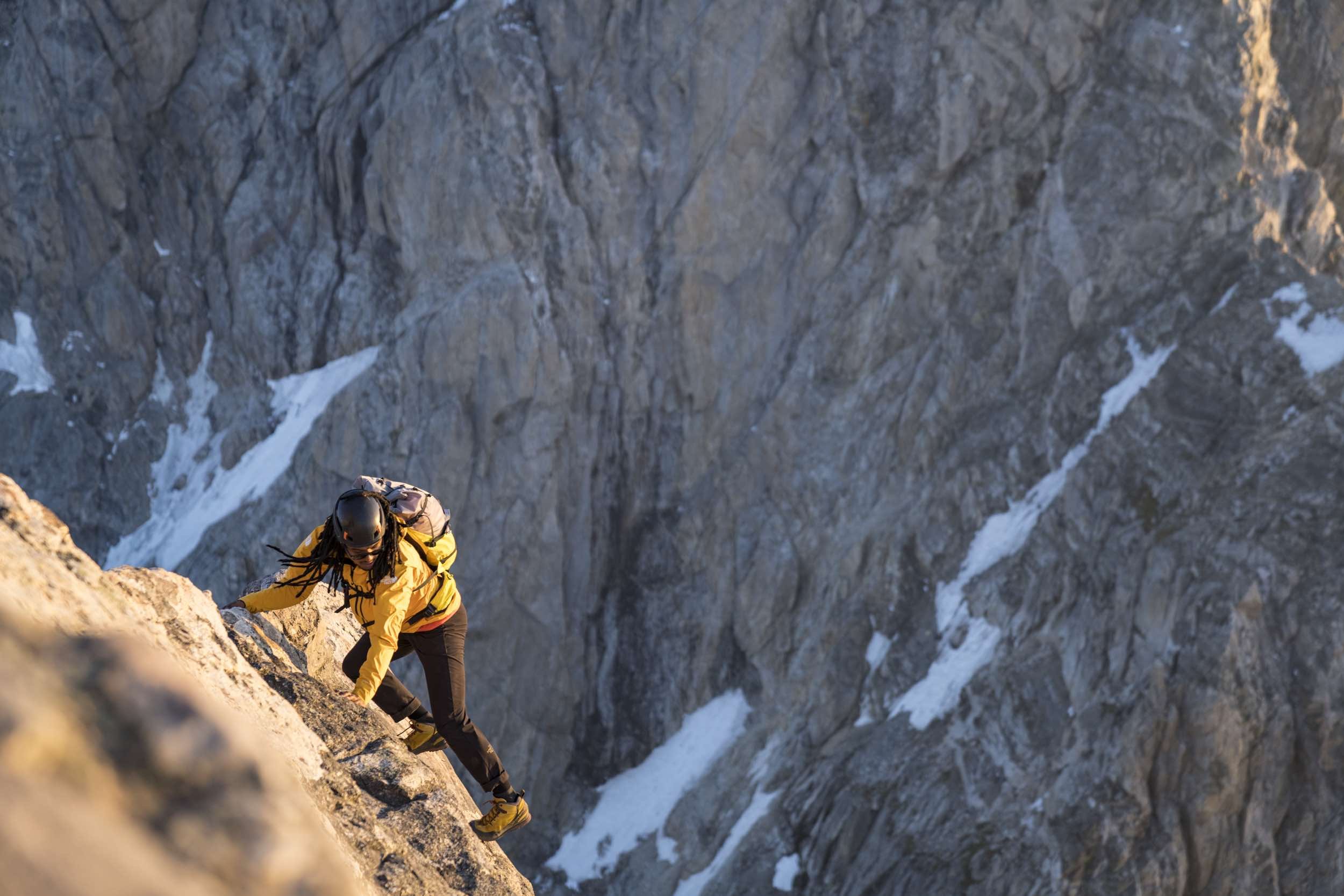The image captures a dramatic bird's eye view from atop a mountain, overlooking a steep canyon below. Dominating the background, a vast gray mountain spans from the top left to the top right of the image, with patches of snow nestling in its ledges and crevices. In stark contrast, the bottom left of the photo reveals a sunlit golden-brown rocky area. Set against this striking landscape, a lone rock climber becomes the focal point. The climber, presumed to be a black male, sports long black dreadlocks that spill out from beneath a black helmet. His attire consists of a bright yellow jacket, brown pants, and sturdy yellow hiking boots. A matching yellow backpack is strapped securely to his back. He is seen gripping the rugged rock face, seemingly unattached to any safety equipment, suggesting he is engaged in a daring freestyle climb. His brown boots are firmly planted, while his hands grasp the rock, conveying both tension and determination in his ascent. The climber's gaze is directed downward towards the ground, further emphasizing the sheer scale and perilous nature of the climb. There is no text in the scene, and the climber is the sole human element in this otherwise vast and silent wilderness.